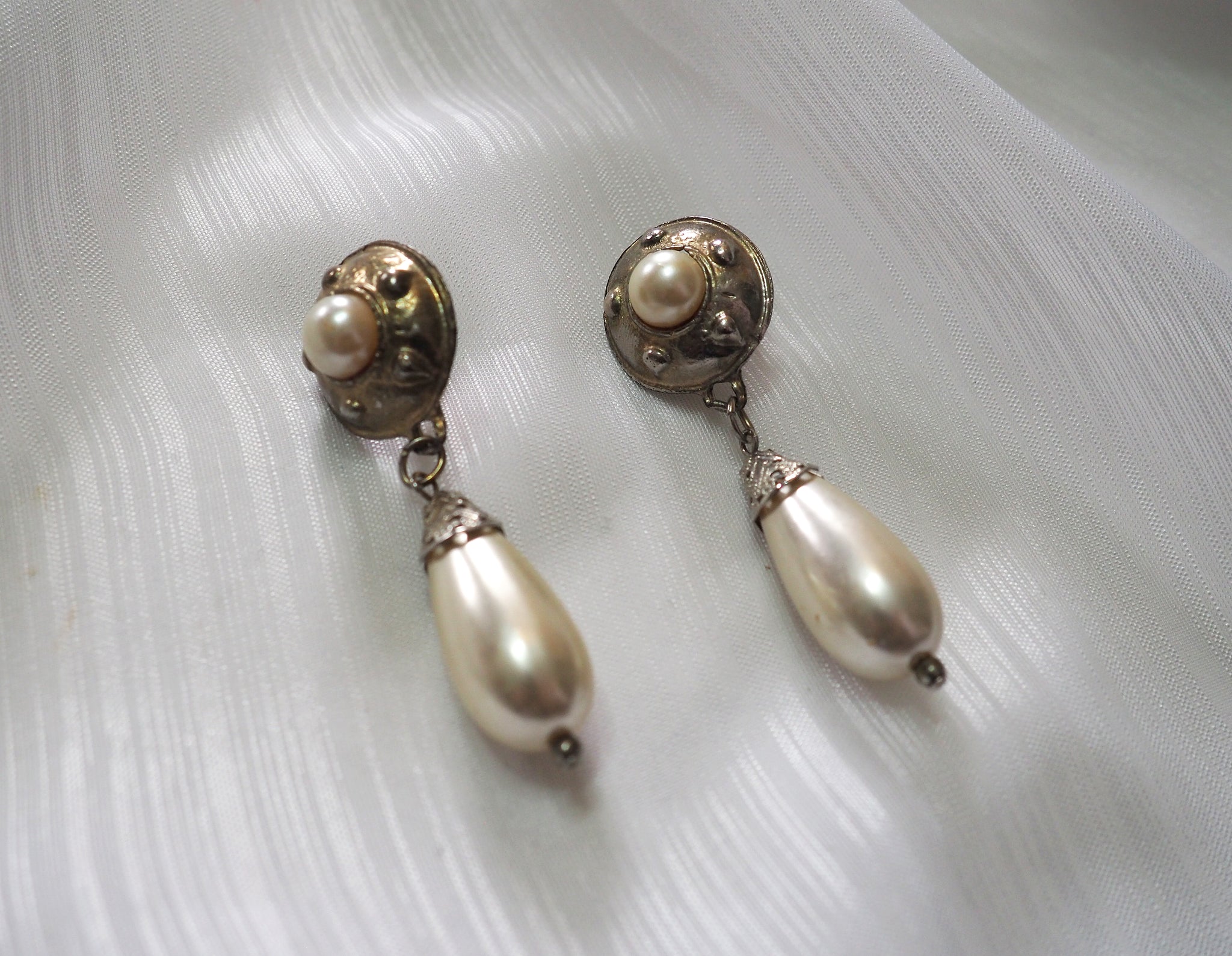The photograph showcases a pair of antique earrings displayed on a silky, white fabric with thin iridescent lines. The earrings feature elongated, teardrop-shaped pearls that dangle gracefully. These hanging pearls are attached to a circular top piece comprised of a gold, dome-like cover embedded with a central pearl. The gold setting is decorated with five small dots, adding intricate detail. These exquisite earrings, linked by a short chain and held by a delicate shaft, capture light beautifully, reflecting their surroundings. The earrings are positioned diagonally from the upper left to the lower right, adding a dynamic composition to the image.